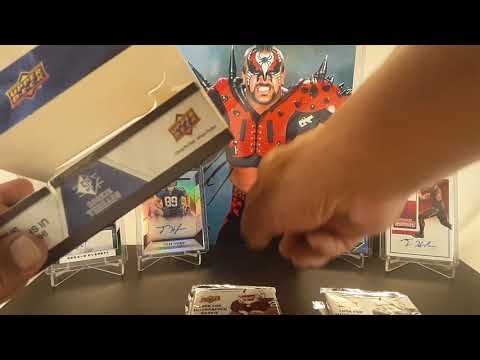In the image, a small black table holds an intriguing collection of sports memorabilia. Dominating the center is an 8x10 cutout of a wrestler clad in highly stylized football gear. His ensemble includes red shoulder pads adorned with black spikes, complemented by red, white, and black face paint featuring a black spider on his white forehead. The wrestler, sporting a mohawk and a fierce expression, stands as the focal point of the display. 

Surrounding the wrestler are multiple clear plastic stands showcasing an array of trading cards. To the left, notable cards include football memorabilia, such as a card of a player wearing a number 89 jersey. On the right side, the exact nature of the displayed cards is ambiguous, potentially featuring basketball players or wrestlers, and perhaps even a depiction that resembles a skier. In the foreground, there are two packs of cards highlighting the diverse collection on the table.

Also in the image, a person's arm extends forward to touch the wrestler's cutout, adding a dynamic element to the scene. Meanwhile, the person's other hand holds a white and blue Upper Deck box, which prominently features gold lettering. This detailed arrangement showcases an eclectic mix of cherished sports items, meticulously arranged on a compact surface.